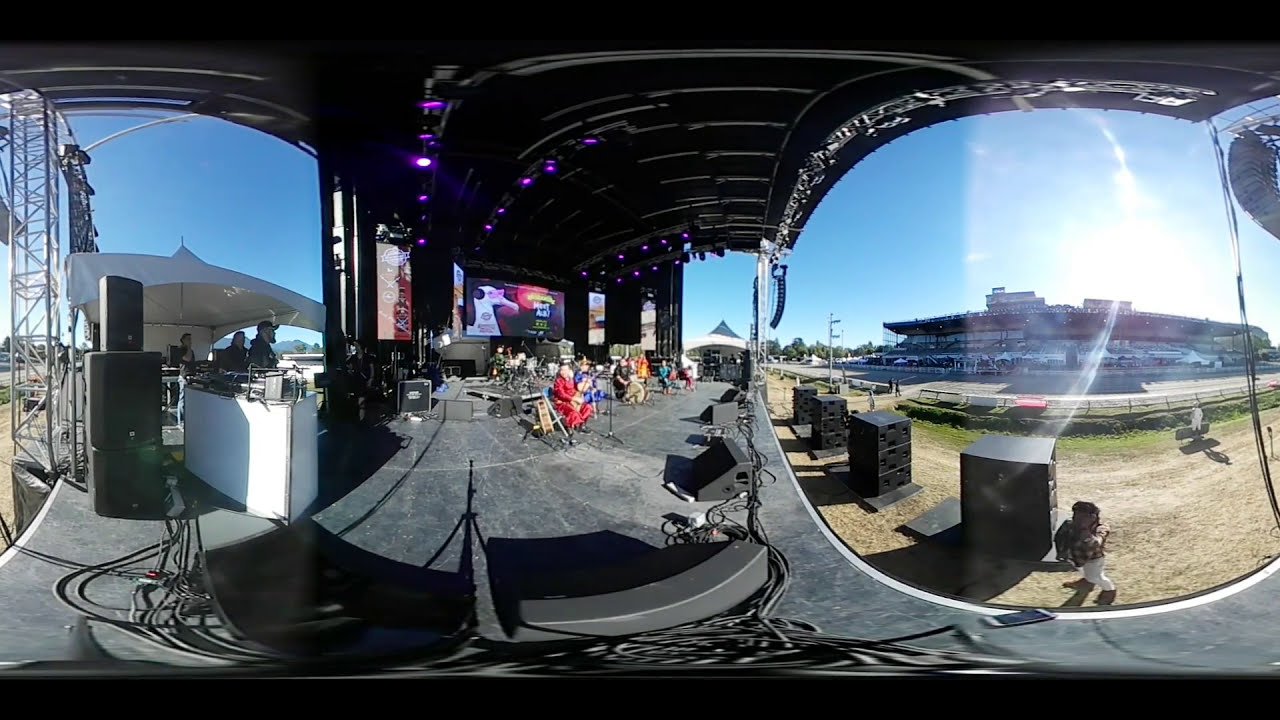The image is a horizontal rectangular photo taken with an unusual lens, leading to a distorted and somewhat unclear view. At the center of the image, there is a stage area featuring various chairs and seated individuals, likely musicians. They are holding instruments commonly used in a band setup, such as guitars, drums, and bass, though this is not entirely clear due to the distance. Numerous cables and pieces of staging equipment including speakers, amplifier cases, and some dark gray floor amplifiers are scattered across the stage. Above them, there are lighting fixtures and screens displaying illegible advertisements.

To the left of the stage, the area extends outdoors where one can see a bright blue sky and several pieces of industrial equipment. Meanwhile, on the right side, there is a view of a grassy and dirt-covered field, with the distant structure resembling a stadium. This field appears to be where the audience would gather to watch the performance. The overall setting is outdoors on a sunny day, possibly during a soundcheck, anticipating a concert or event later in the day. The color palette includes shades of black, white, gray, red, blue, turquoise, and purple.